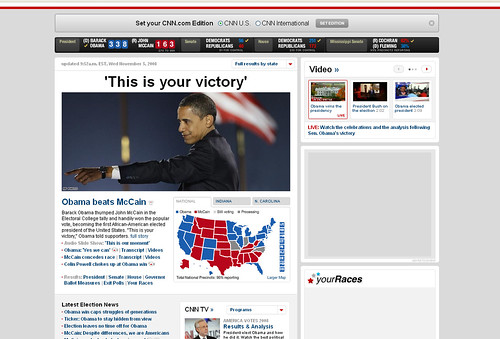The image depicts a webpage from CNN.com, distinguished by a gray-themed background indicative of a news article format. At the top, the page features a banner labeled "Set Your CNN.com Edition," with options for "CNN US" and "CNN International," accompanied by a gray "Set Edition" button. Below, a black bar presents an advertisement related to the presidential race between Barack Obama and John McCain.

Central to the page is a prominent headline reading "This is Your Victory," with a subheader stating "Obama Beats McCain." The text below the headline is somewhat illegible due to low resolution. Adjacent to the text is a U.S. map colored in red and blue, highlighting the states that flipped in favor of either candidate during the election.

Beneath the main article, a section titled "Latest Election News" features numerous blue-highlighted links to various articles. On the right side, the page includes segments labeled "CNN TV" and "Video," with the latter showcasing three video previews.

A notable element is a photograph situated under the "This is Your Victory" headline, depicting Barack Obama pointing towards the crowd, likely captured during his victory speech. The overall webpage capture highlights key elements of CNN’s coverage during the 2008 presidential election.